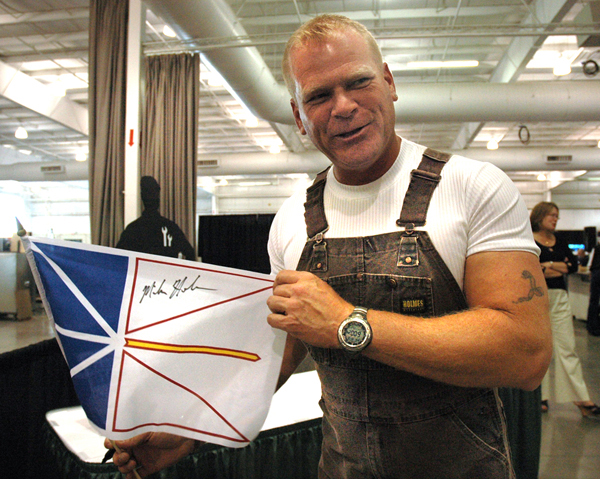In the image, renowned real estate expert and television personality Mike Holmes is captured smiling and proudly holding a small flag featuring a blue and white design with bits of red and a yellow stripe. The flag also displays a signature in the top right triangle, indicating a recent autograph. Holmes, known for his short blonde hair and ruddy complexion, is dressed in brown dungaree overalls over a tight white t-shirt, showcasing a scorpion tattoo on his left bicep and a prominent watch on his left wrist.

The setting appears to be an office or industrial space, characterized by a white ceiling with fluorescent lights and visible large industrial pipes. The shiny, grey-tiled floor and beige curtains clumped to the sides add to the clean and well-lit ambiance. In the background, a woman in a black shirt and white pants is visible, engaged in conversation, underscoring the professional environment.